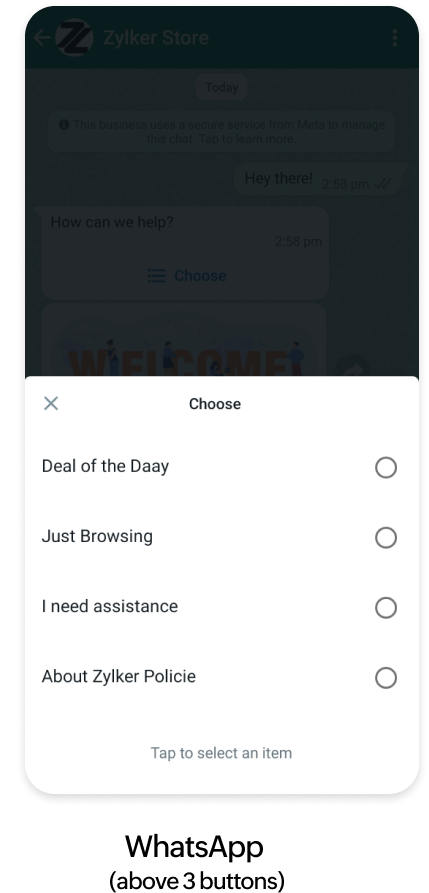The image depicts a screenshot of an app interface. A semi-transparent, dark-tinted overlay focuses attention on a prominent white pop-up menu located at the bottom of the screen. At the top of the pop-up, a message reads "Choose," flanked by an "X" button on the left. Beneath this, four vertically listed button options are available: "Deal of the Day," "Just Browsing," "I Need Assistance," and "About Zilker Policy." Each option has a circular button to its right for selection. Below the buttons, instructions state "Tap to select an item." The underlying app can still be vaguely seen through the dark tint, displaying the heading "Zilker Store" with what appears to be a chat window. At the bottom of the phone screen mock-up, the word "WhatsApp" is visible above three additional buttons.